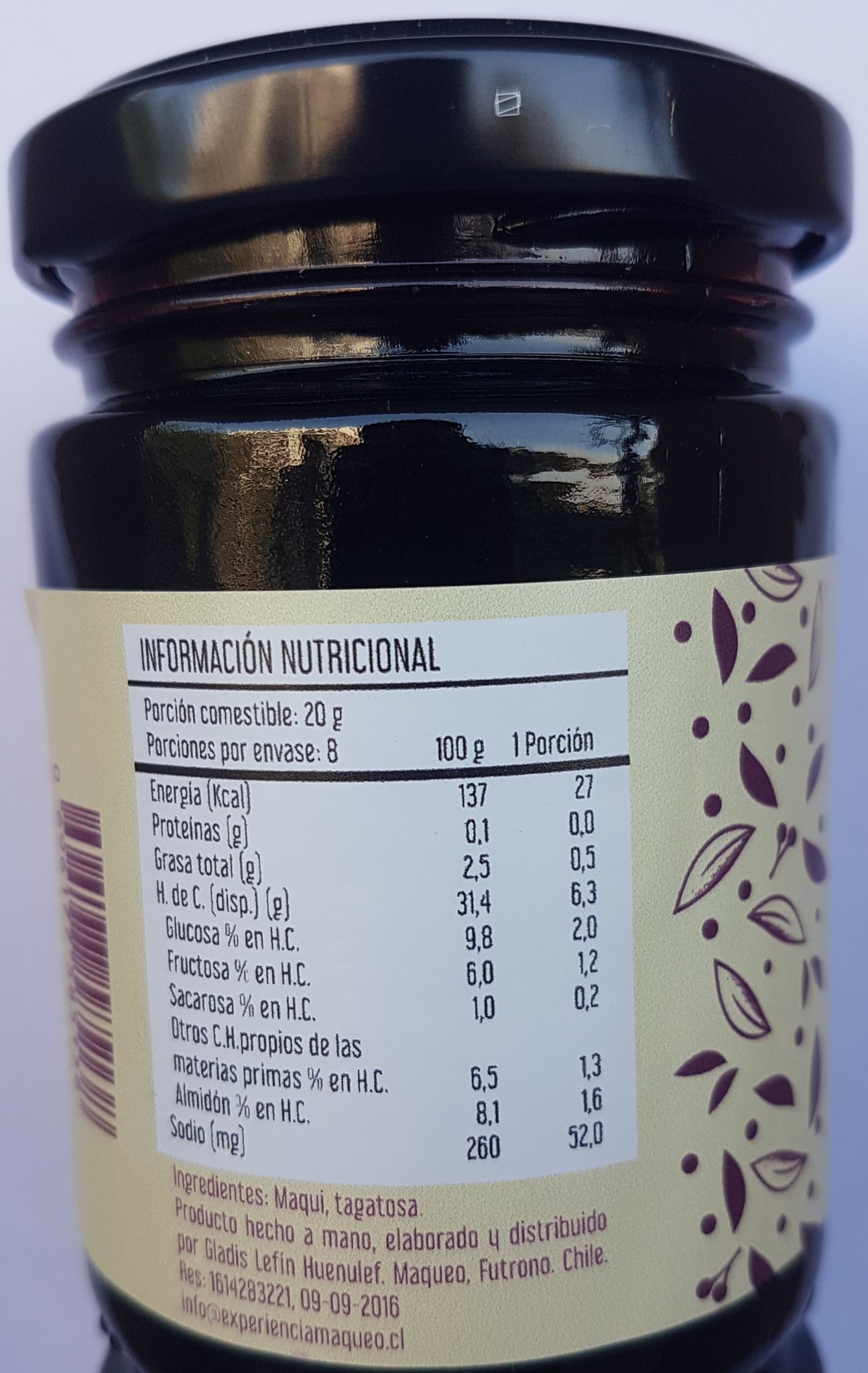The image depicts a black, shiny plastic bottle, reminiscent of glass, featuring an off-white label. This label includes detailed nutritional information in another language, likely Spanish or Portuguese. The label provides data for 100 grams and one portion, including calories (kcals), proteins, fats, glucose, fructose, sucralose, sodium, and other substances like uric acid and ammonium. The label also lists ingredients, which appear to be in Spanish, with words like "Chile." The label is adorned with purple leaves and features a purple barcode on the left side. The lid of the bottle has a white mark characteristic of plastic. Additional details on the label include a resource number (161428321) and a date (09-09-2016), with contact information from "EXPERIENCIAMAQUEO.CL."